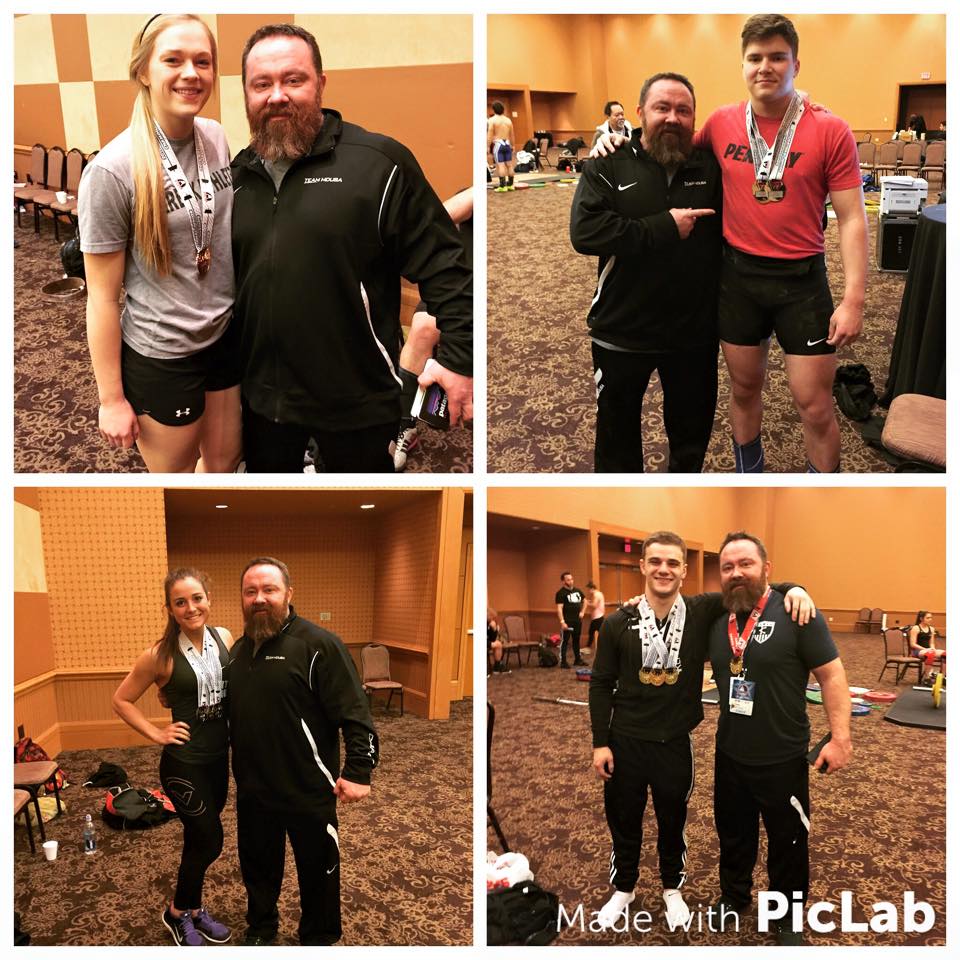This detailed collage features four distinct photos, each of which includes a common figure: a shorter, burly man with a brown beard, clad in a black Nike tracksuit with white trim. In the upper left image, he poses with a tall, blonde woman wearing a gray shirt and black shorts, both adorned with medals around their necks. They stand in a convention center room decorated in shades of tan and cream with checkered walls and chairs lining the background. The upper right image depicts the same man with a significantly taller, younger gentleman dressed in a red shirt and black shorts, showcasing two medals around his neck amidst a similar backdrop of chairs and plain tan walls. The bottom left photo captures him with a petite woman in a green tank top, black yoga pants, and many medals (at least three to four), set against the same conference room's perforated boards and checkered wall patterns. Finally, in the bottom right image, the burly man is seen beside another man of equal height, who sports a black long-sleeve shirt, track pants, and three medals, with 'Made with PicLab' watermarking the photo in white font at the bottom right corner. The room features consistent carpeting and shades of creamy white and dark tan, emphasizing the uniform setting across the images.